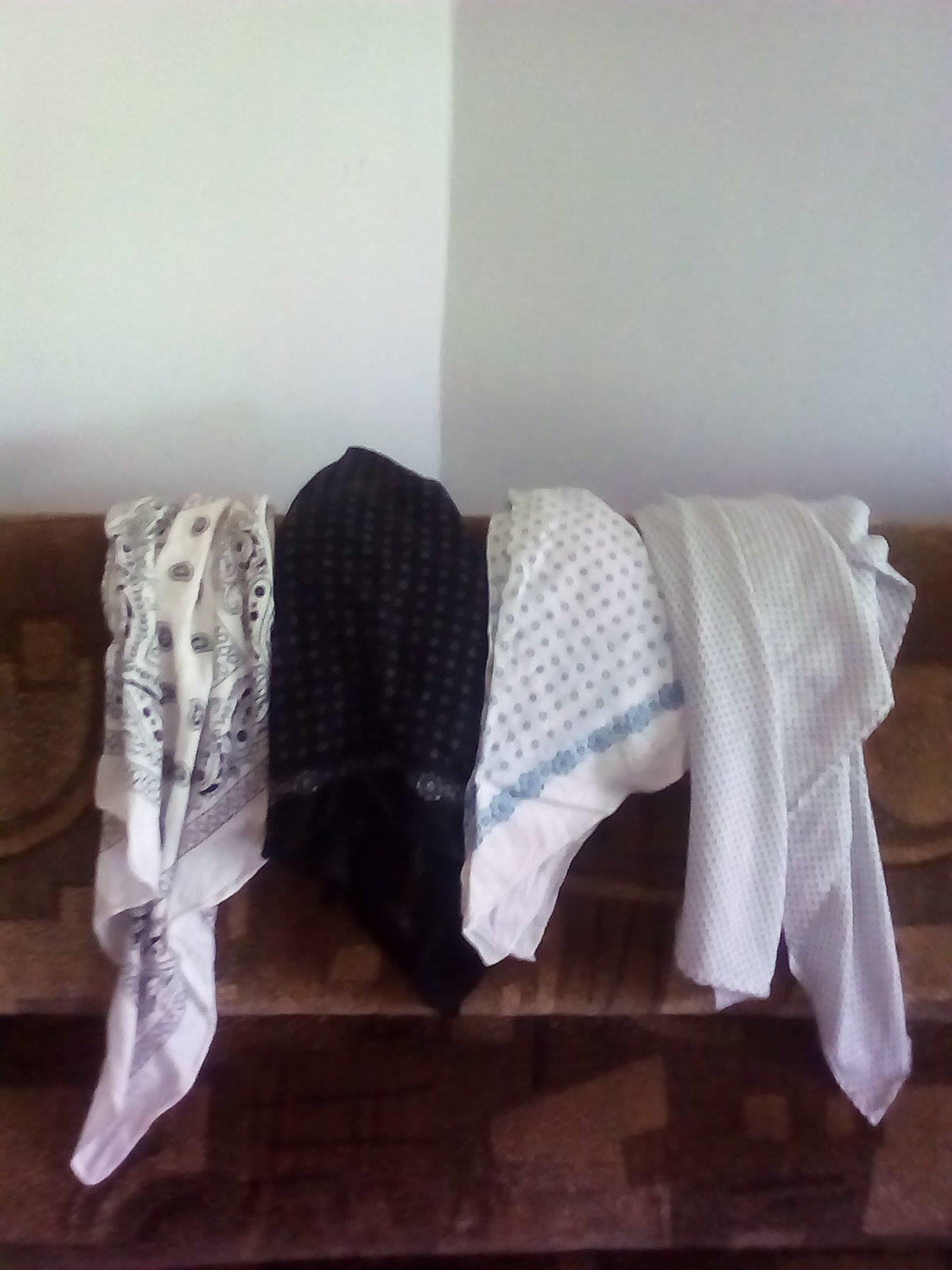The photograph captures a corner of a room where white and greyish walls meet at an angle in the center of the image. Positioned below this, taking up almost the entire width of the photo, is a piece of brown wooden furniture, possibly a dresser or a storage container, with a subtle ledge under the clothing items. Draped over this wooden piece are four different articles of fabric arranged with their corners facing downward.

From left to right, the first fabric is a white bandana marked with a black paisley design, slightly wrinkled and folded such that you can see both its border and center motifs. The second item is a solid black piece with a subtle pattern of small white squares, indicating a possible border design. The third is a triangularly folded white bandana, featuring a light blue floral border and tiny floral prints inside the border. The fourth item is an off-white, textured fabric that lacks any decoration, resembling more of a shawl, and appears casually placed. The fabrics are neatly arranged yet maintain a casual, slightly scrunched appearance, enhancing the composition's authentic feel.